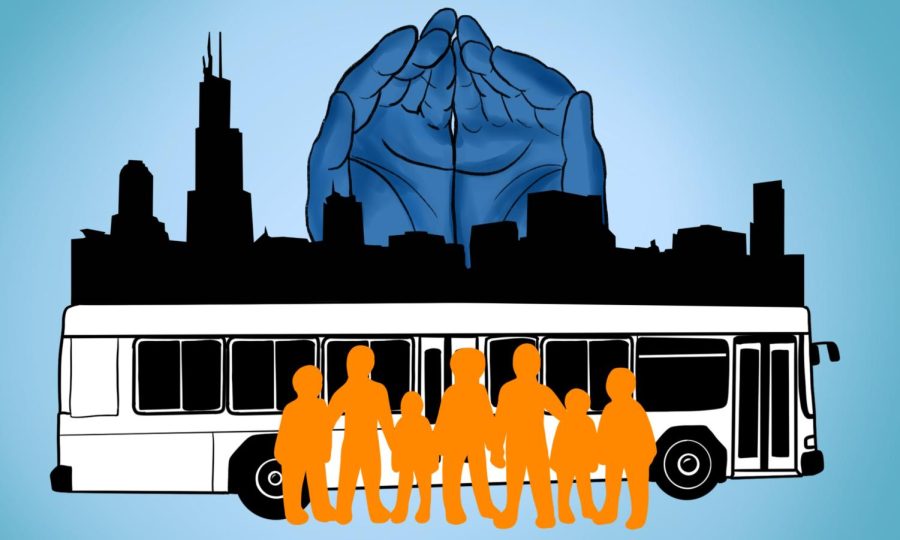The image depicts a vibrant city scene characterized by a diverse array of elements and a striking color palette. Central to the artwork are seven orange silhouettes of people, appearing to be a mix of adults and children, standing together in front of an elongated, black and white bus. These figures, prominently outlined in orange, draw immediate attention in the foreground. Directly behind the group, the bus itself stands as a significant centerpiece of the scene, depicted in stark contrast with its black and white color scheme. 

Further into the background, an intricate silhouette of downtown buildings spans across the horizon, rendered in solid black against the predominantly light blue sky, conveying the essence of an urban skyline. Above these buildings, a pair of dark blue, clasped hands rise against the light blue backdrop, seemingly cupped as if holding something precious or symbolizing unity and support. This complex layering of silhouettes and colors – the orange figures, the monochrome bus, the black cityscape, and the blue hands – coalesce to create a visually compelling and evocative imagery indicative of communal harmony within an urban setting.